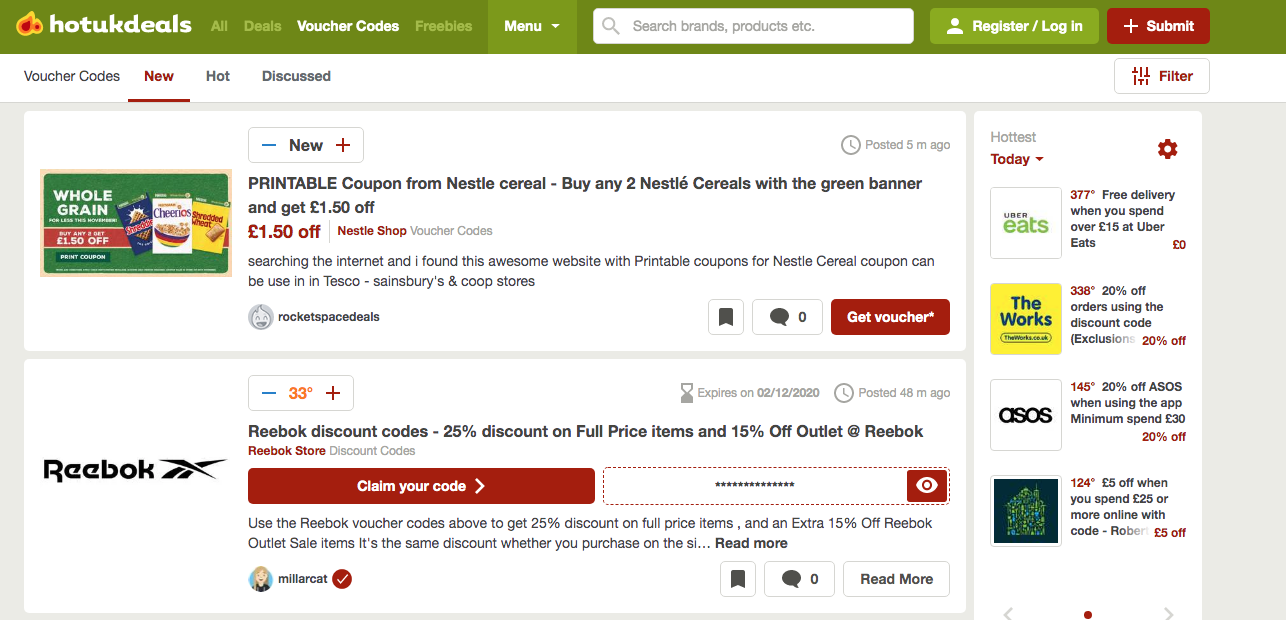Below is a cleaned-up and detailed descriptive caption based on the provided voice transcription:

---

The image showcases a vibrant webpage adorned with a dynamic flame icon labeled "Hot UK Deals." The header features navigation buttons such as "All Deals," "Voucher Codes," "Favorites," "Drop Domain," "Search," "Brands," and "Products." To the right, there are options for users to "Register/Login" and a "Submit" button. 

Underneath, a series of tabs labeled "Voucher Codes," "New," "Hot," "Discussed," and "Filter" provide further navigational assistance. 

On the left sidebar, there's a prominent green section featuring various icons. Encased in boxes, trails, and buttons, there are highlighted offers like "£150 Off" and a "Printable Coupon for Nestle Cereal." One of the promotions reads: "Buy any two Nestle Cereals with a green banner and get one free." 

Additionally, there are mentions of Nestle Codes, Shop, Voucher Codes, Search Engine, and other categories like Funds and Hospital. The Nestle cereal coupon is specifically usable at Tesco, Sainsbury's, Co-op, and other listed retailers. 

Highlighted deals include a "Drop is the hardest to lay, 377 degrees," and another offering "Over £15 off Air Breeze." There’s also mention of discounts such as "33 Degrees" and "21% off ASOS," suggesting substantial savings.

---